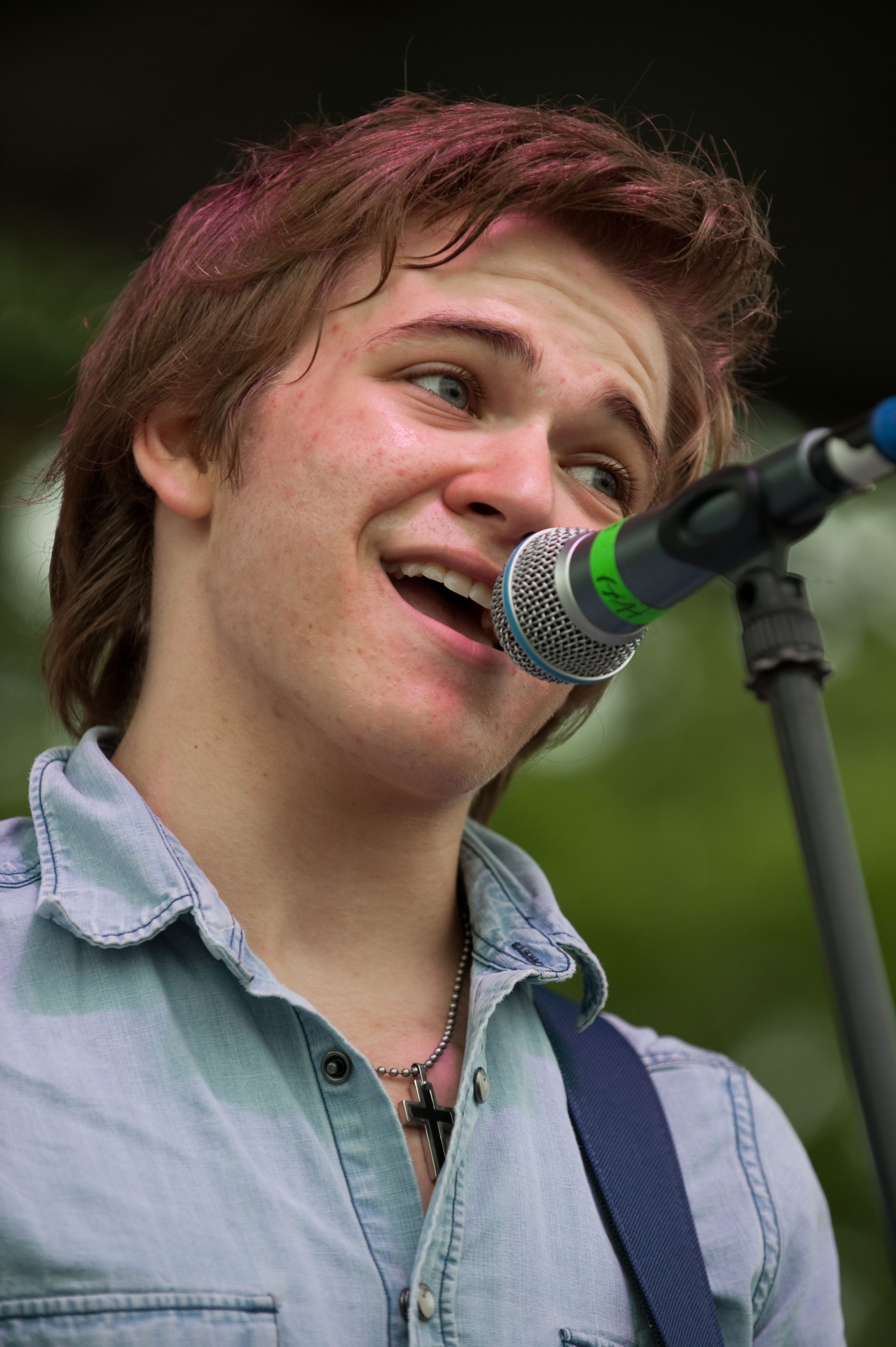In the image, a young pop singer with expressive features and slightly long, brown hair, possibly tinted with red or purple, is captured mid-song, with his mouth open as he sings into a microphone. The microphone has a distinctive green stripe around it and is mounted on a metal, gray stand. He’s looking off-frame to the right and slightly upward. Dressed in a blue jean jacket with visible buttons and a blue guitar strap slung over his shoulder, the singer also wears a black enameled cross necklace. The background appears to be outdoors, with blurry trees behind him. His face, framed closely from the mid-chest up, might show signs of eczema.